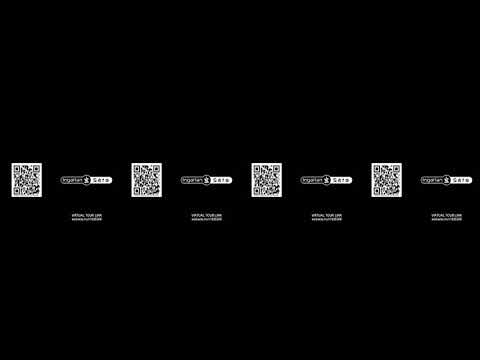The image displays a solid black background with four evenly spaced, white and black QR codes arranged horizontally across the center. Each QR code is separated by a horizontal capsule-shaped insignia, featuring very small, illegible text. Below each insignia, there is a soft, blurry white lettering that appears difficult to decipher. The overall composition, with the stark contrast of the white QR codes and inscriptions against the black backdrop, suggests it might be an advertisement or an attempt to draw attention, although the exact purpose remains unclear.